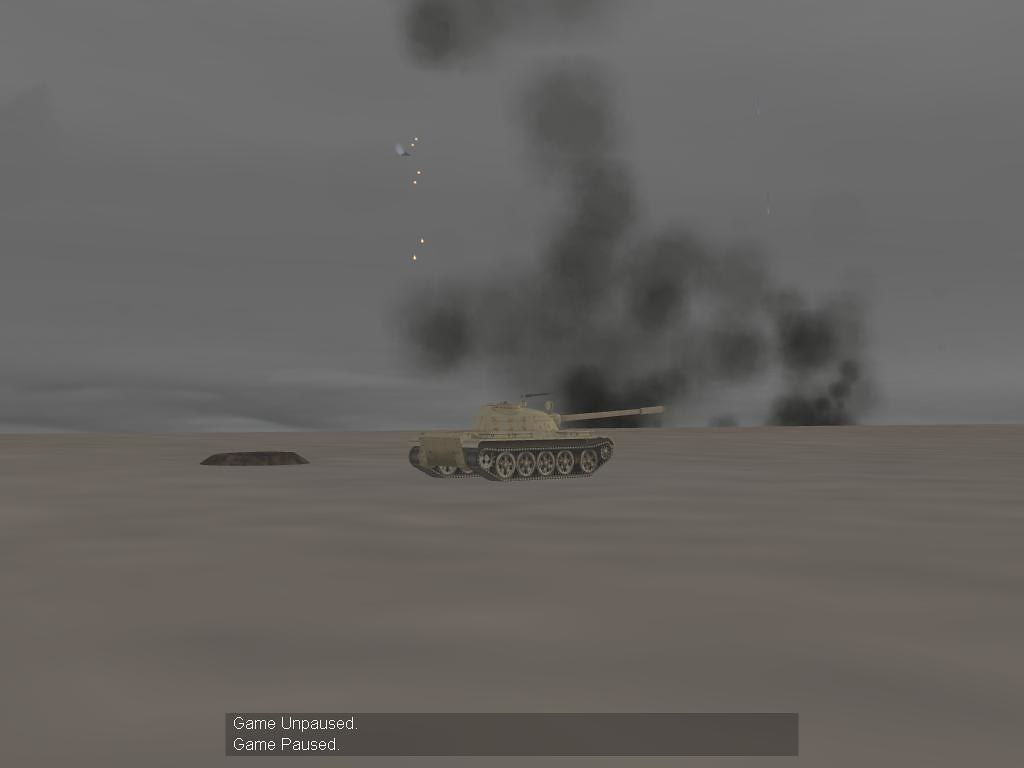Screenshot from a video game showing a grayish-brown ground in the foreground. Dominating the scene is a tan-colored tank positioned towards the back, with its large turret and weapon aiming to the right side of the image. The background is filled with dark gray smoke, adding a sense of chaos and tension. Bright yellow dots punctuate the smoky sky, creating a stark contrast against the very light gray backdrop. At the bottom of the screenshot, there is a dark gray rectangular box containing white text, first displaying "Game Unpaused" and below it, "Game Paused," indicating a transition within the gameplay.